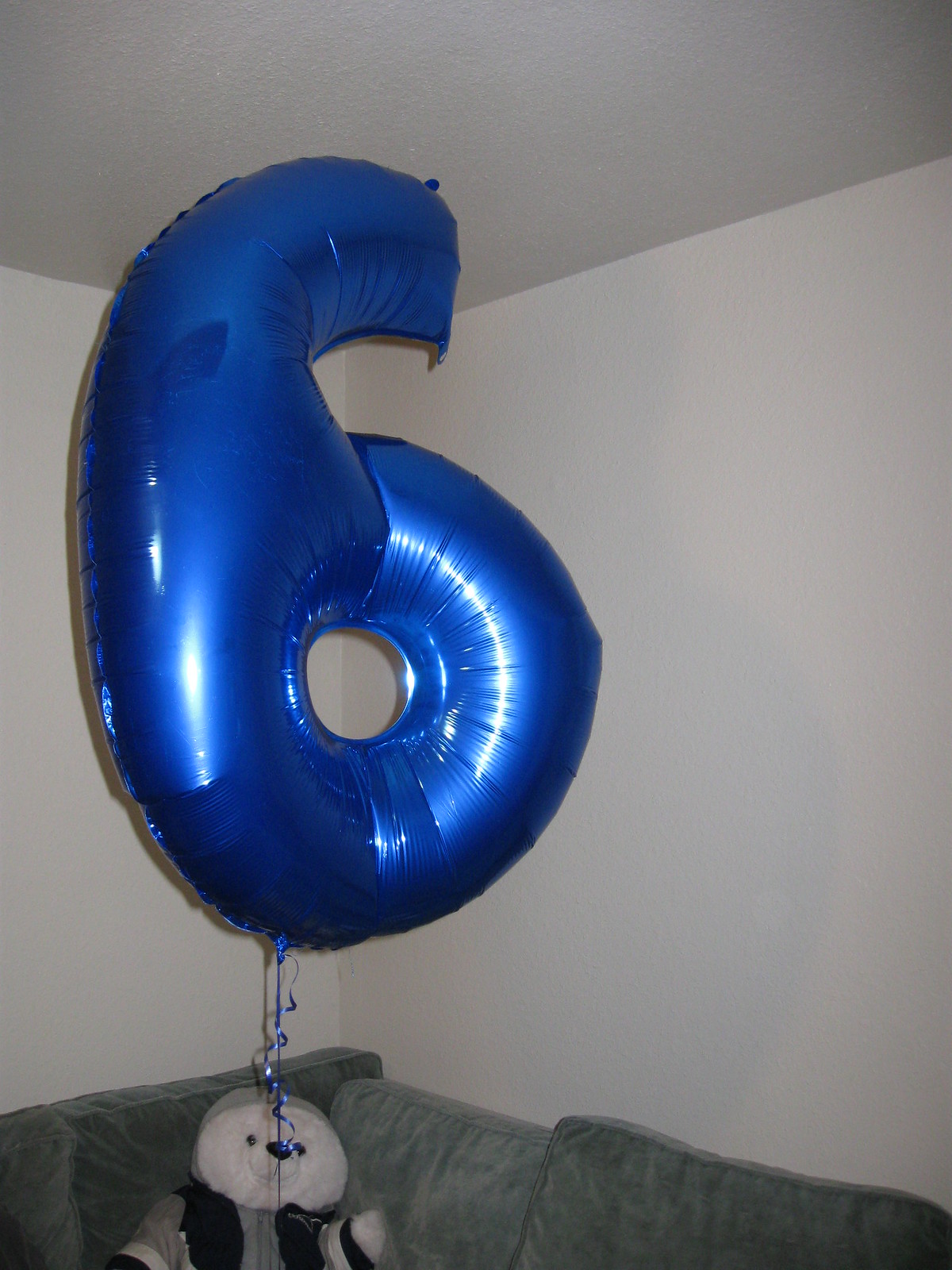This close-up photo captures a giant Mylar balloon in the shape of the number 6, positioned in the corner of a white room. A blue ribbon holds the helium-filled balloon in place, with another curled ribbon dangling at the bottom. The balloon casts a shadow behind it, creating an illusion of a black outline. Light reflections on the balloon produce shiny spots and white lines along its surface.

Below the balloon, a gray couch is partially visible, adorned with cushions. A white teddy bear dressed in a gray, black, and white shirt sits on the couch. The photograph also shows the point where the room's white walls and ceiling converge.